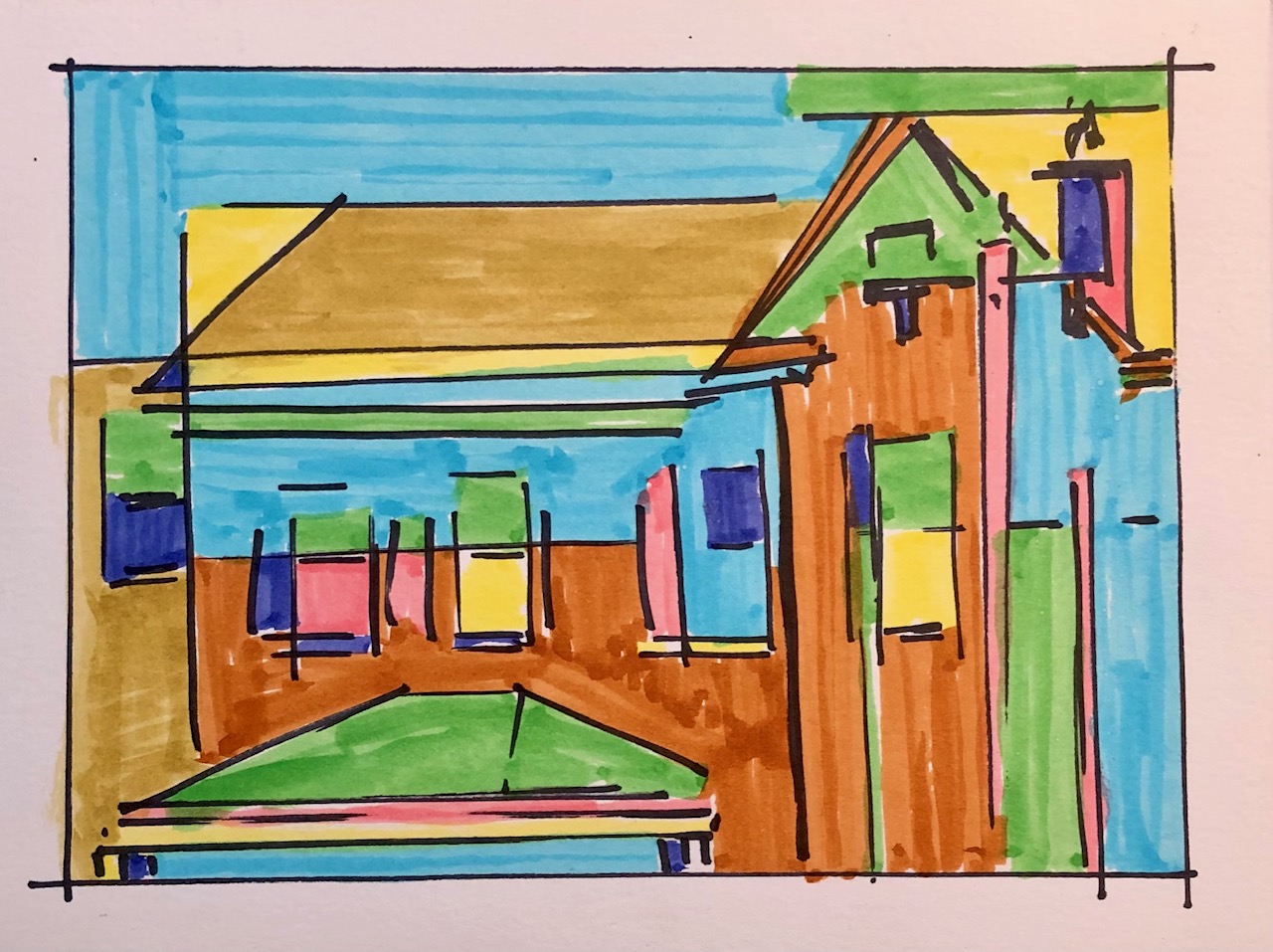This image features a low-poly, abstract-style house rendered in vibrant, non-traditional colors. The house's structure is adorned with a brown roof that includes splashes of yellow and blue, adding to its unique aesthetic. Yellow windows and a yellow doorway contrast against the multicolored walls, which incorporate shades of green and brown. The driveway in front of the house is a striking green, setting a vivid tone. A heavily marked brown area forms the foundation beneath the house. The entire scene is set against a bold, pink background, enhancing the overall playful and artistic nature of the composition.